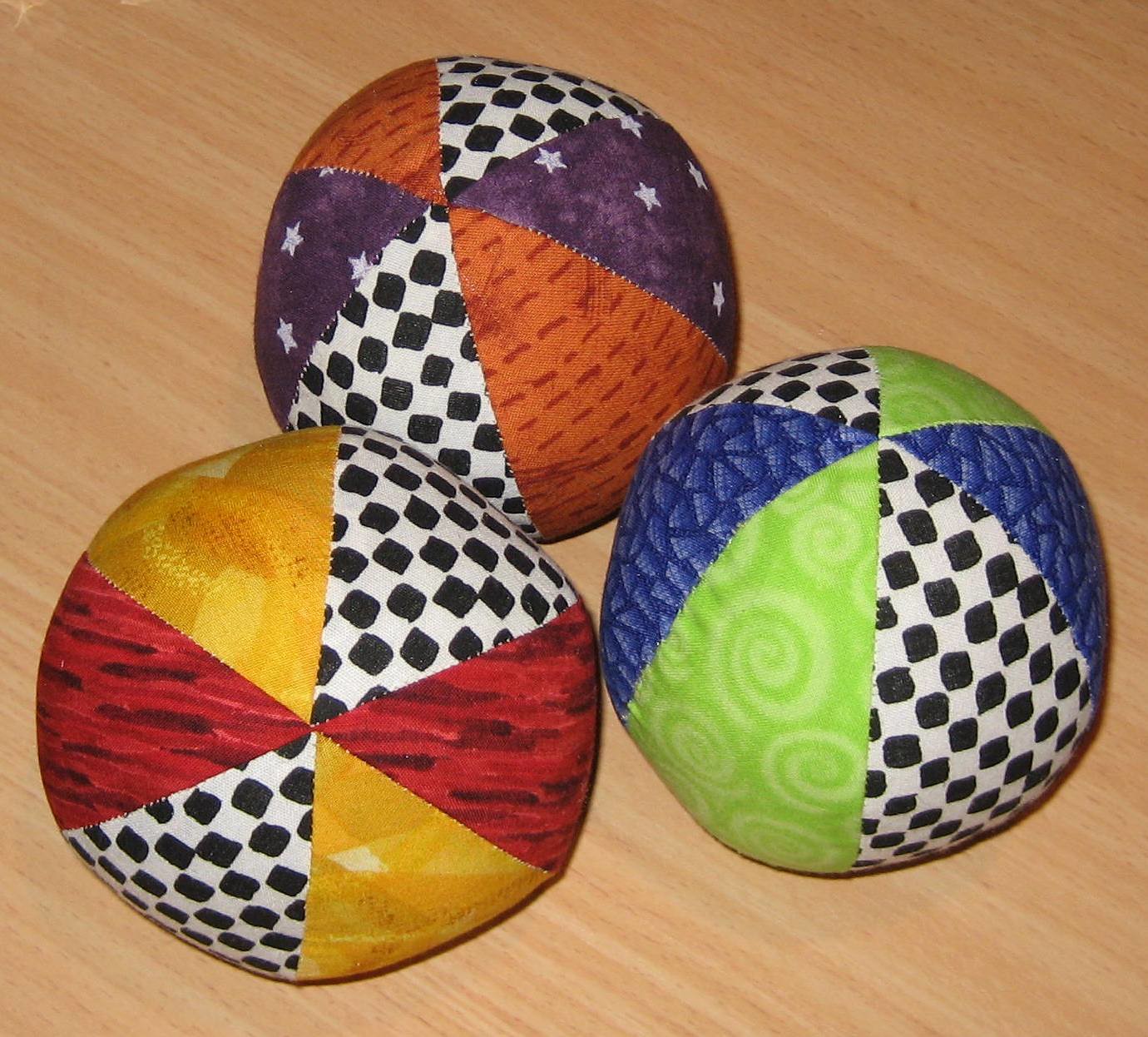On a light wooden tabletop, three hacky sack balls are arranged in a triangle. Each ball is decorated with a distinct set of vibrant panels, including a shared black and white checkerboard pattern. The first ball features two purple sections adorned with white stars, two orange sections with darker rust-colored stripes, and two black and white checkerboard sections. The second ball has two checkerboard sections, two gold sections, and two red sections with black stripes. The third ball showcases two checkerboard sections, two blue sections with light blue triangles, and two green sections with light green swirls. The balls appear soft, similar to bean bags or Nerf balls, and are detailed with intricate designs that meet at their peaks, forming a symmetrical pattern.